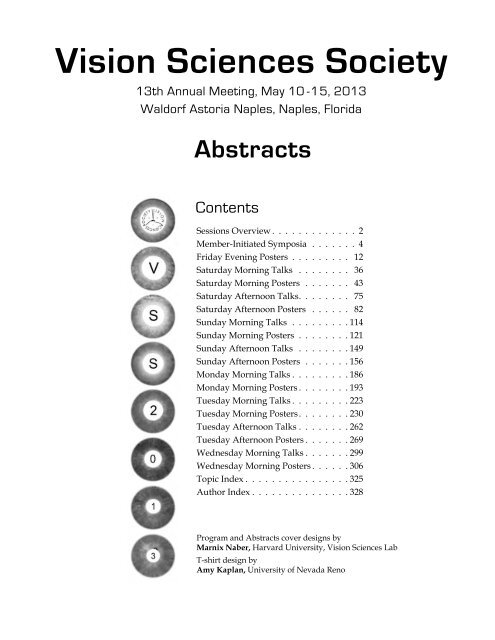The image is a detailed page displaying the table of contents for the Vision Sciences Society's 13th Annual Meeting, held from May 10-15, 2013 at the Waldorf Astoria in Naples, Florida. The page prominently features the meeting title in bold black letters, with subheadings listing various events and sections such as Sessions Overview, Member Initiated Symposia, Friday Evening Posters, and multiple sessions of Morning and Afternoon Talks and Posters organized by day—from Saturday to Wednesday. At the bottom of the page, credits include the Program and Abstracts Cover Designs by Marnik's Neighbor of the Harvard University Vision Sciences Lab and T-Shirt Design by Amy Kaplan from the University of Nevada, Reno. To the left of the table of contents, there is a stack of eight spherical objects resembling pool balls. These spheres are labeled with the letters "VSS" and the year "2013," with the topmost sphere featuring a design similar to a Mercedes logo.